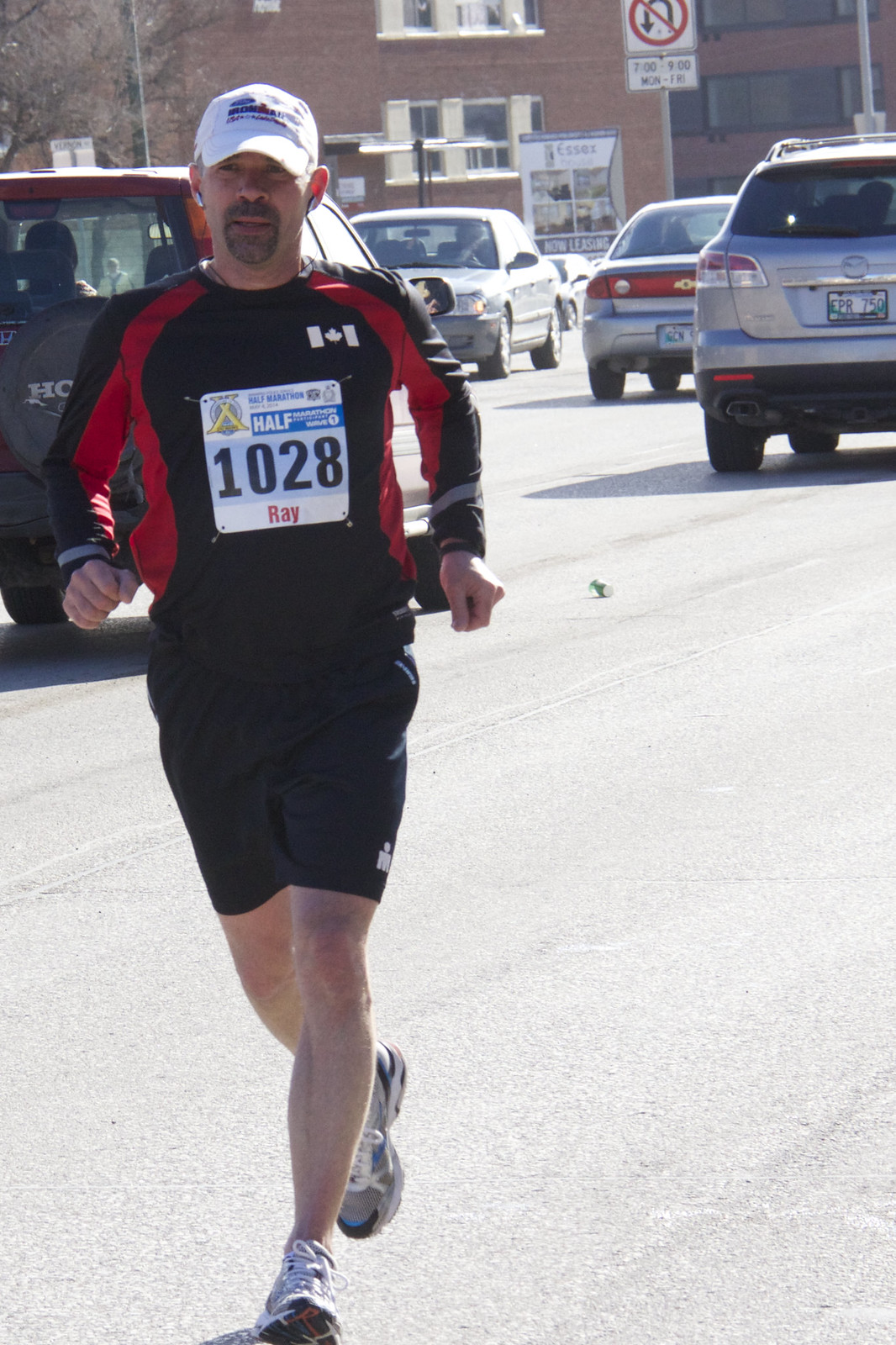In this brightly sunlit photograph, a Caucasian man with a mustache and goatee is captured mid-run on a gray asphalt street. He is participating in a race, as indicated by the bib pinned to his black and red long-sleeve shirt, displaying the number 1028 and the name "Ray." The shirt features red stripes along the sides of the torso and undersides of the sleeves. Ray is also wearing black shorts, gray and white sneakers with blue and black trim, and a white baseball cap with some lettering faintly visible. Behind Ray, to the left, a diagonal line of cars continues towards the upper right corner of the image, enhancing the sense of depth. The distant background shows a faded dark red brick building with windows and a traffic sign reading "No U-Turns, 7 to 9, Monday to Friday." Shadows indicate it's a sunny day, contributing to the clear, vibrant details of the scene.